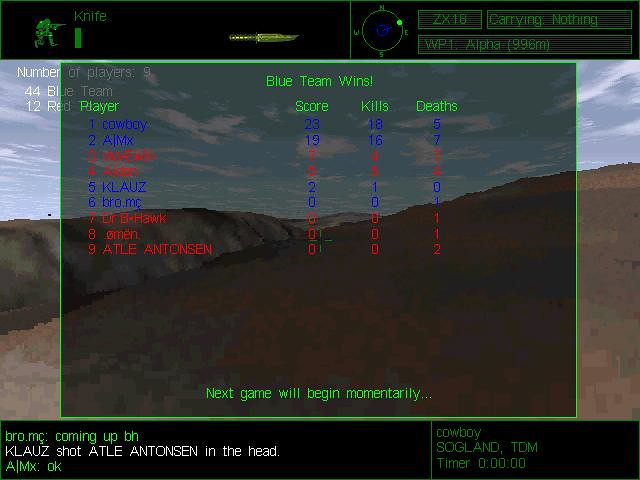This image is a screenshot from an old-school first-person shooter game, likely from the early Windows XP era, showcasing a pixelated and low-resolution graphic style typical of that time. The scene features an outdoor landscape with rolling brown hills and a grayish-blue cloudy sky. Dominating the center is a grayed-out scoreboard with green trim, listing nine players along with their kills, scores, and deaths. At the bottom of this box, green text announces that the "Next game will begin momentarily." The upper section of the screen includes two black horizontal bands; the top one shows an outline of a kneeling soldier next to the word "knife" and an image of a knife, suggesting the player's current weapon. The upper right corner contains a circular map for player positions, along with other game-related information. The lower black band features a chat screen on the left and a timer set to zero on the right, indicating the conclusion of a match.